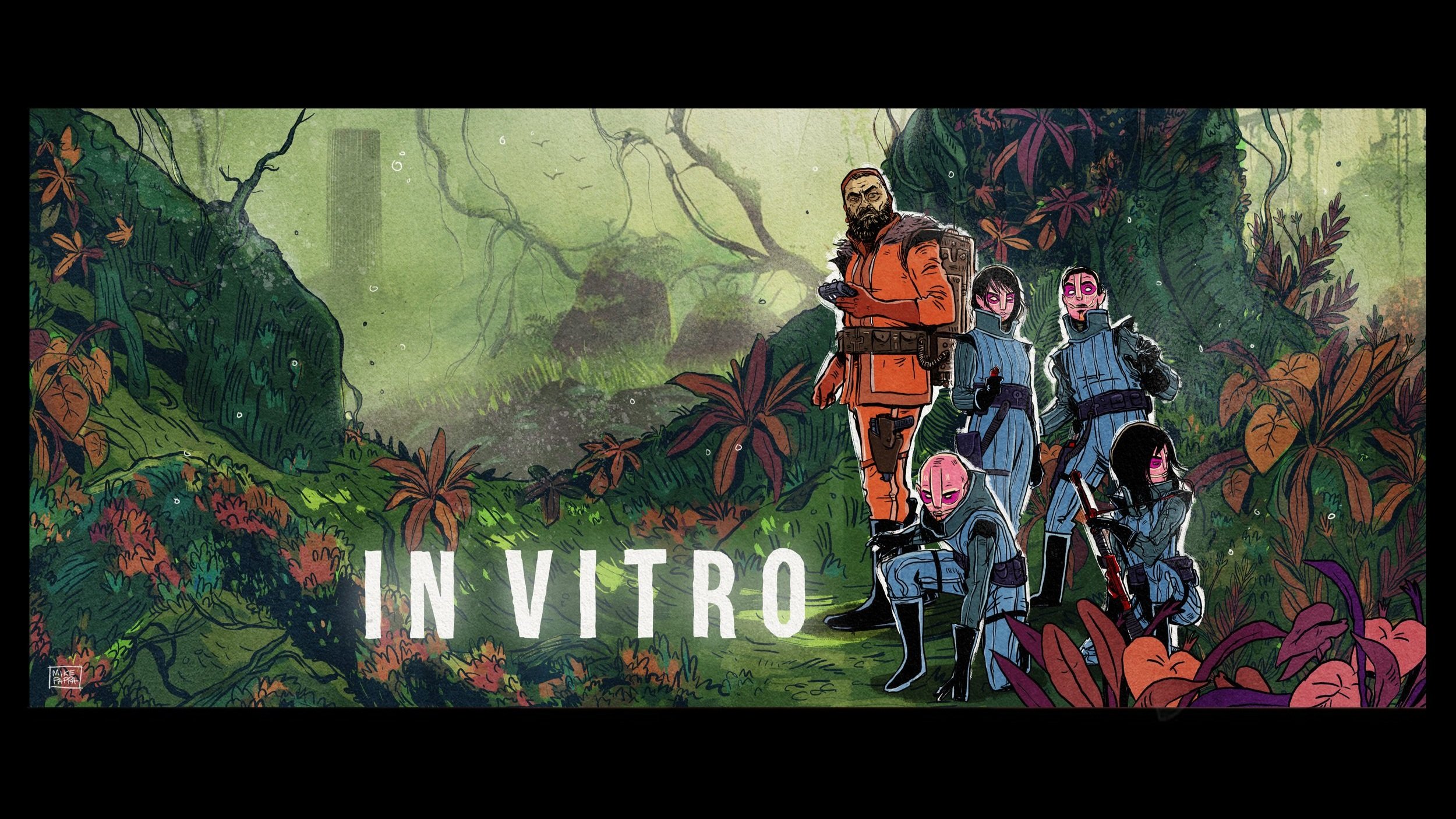This intricate illustration, seemingly from an animation or video game, portrays a diverse group of space travelers in an extraterrestrial jungle shrouded in mist. The image features four aliens in blue space suits, characterized by their humanoid form, lack of pupils, and pinkish areas around their eyes. Beside them stands a taller human in an orange space suit and backpack, suggesting a leadership role. Set against a backdrop of vibrant orange and purple plants, trees, and rocks, the group appears to have just arrived in this enigmatic fantasy land, evidenced by two aliens squatting and holding what seem to be futuristic weapons. Central to the image are the white letters "In Vitro," emphasizing the title and tying the scene together with a sense of mystery and adventure.